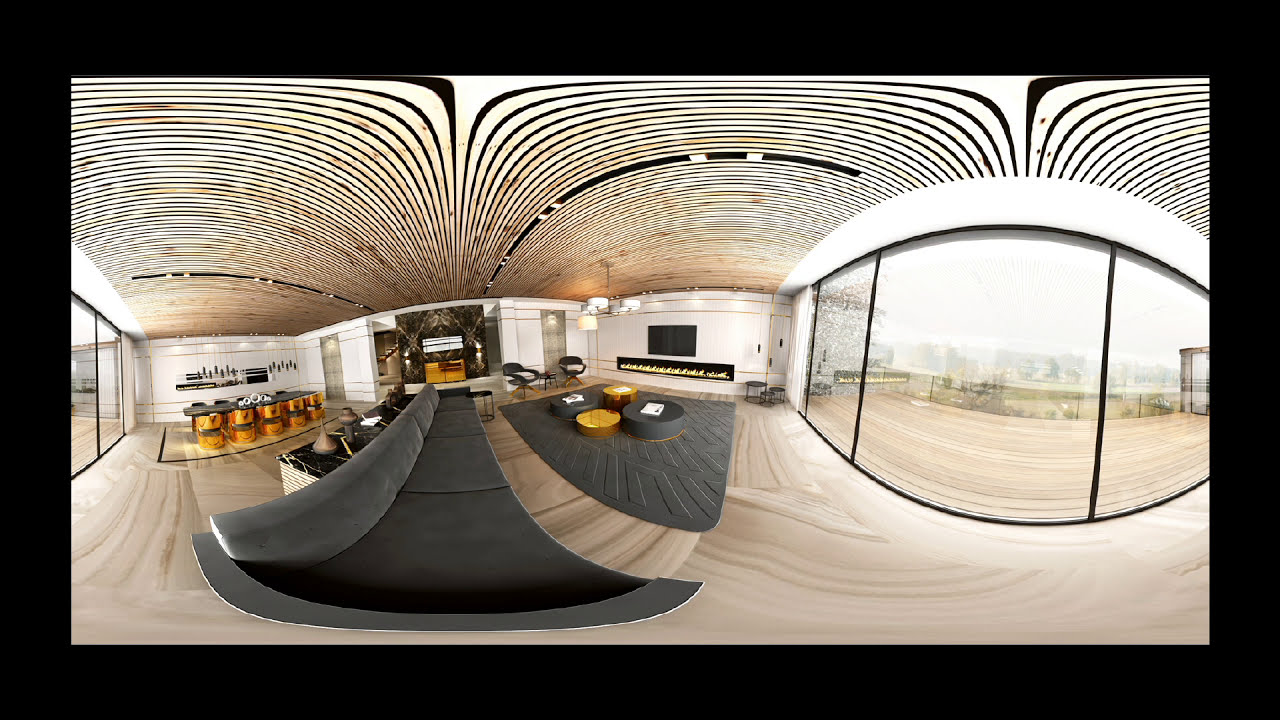This horizontal-rectangular image, taken with a special panoramic lens, displays an office interior that's dramatically distorted, causing abnormal curvature. The room features a prominent floor-to-ceiling, three-paneled window or sliding door on the right side, viewed as an oval shape due to the lens. Black and white stripes stretch across the ceiling, resembling zebra stripes, and continue onto the opposite wall, which is also lined with windows. 

In the left half of the image, a large gray couch emerges with visible distortion, accompanied by several small coffee tables on a gray area rug. The center of the image, challenging to interpret due to the curvature, appears to contain a mounted TV and sound bar on a white wall, possibly above an artificial fireplace. The entire image is framed by a thick black border, adding to its unique, almost surreal perspective. The floor, resembling wood tiles, extends across the scene, leading up to what might be a pulpit or lectern in the background.